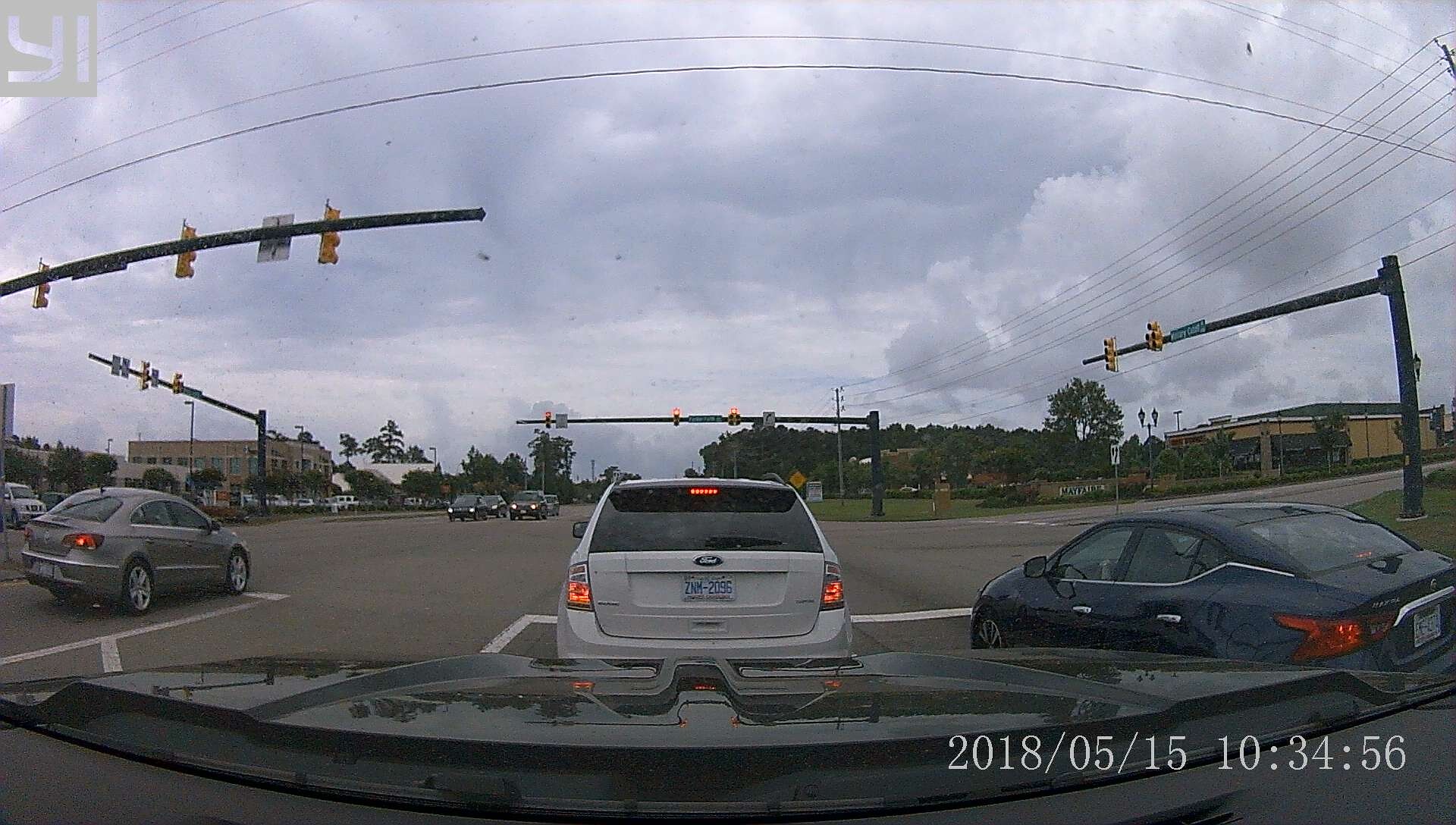The photograph captures a scene from inside a vehicle, clearly showing the vehicle's front end. Dominating the center of the image is a white Ford SUV, positioned slightly lower than the center. To the right of the SUV, a blue car is visible, while on the far left side, a grayish car can be seen. All three vehicles are waiting at a red stoplight, which is situated in the background. Below the stoplight, cars moving in the opposite direction can be noticed. The scene is framed by buildings on both the left and right sides, with numerous trees adding a natural element to the urban setting. The sky above is filled with hazy clouds, lending a somewhat overcast atmosphere to the image. In the bottom right corner, there's a timestamp and date in white, adding a detailed touch to the snapshot.